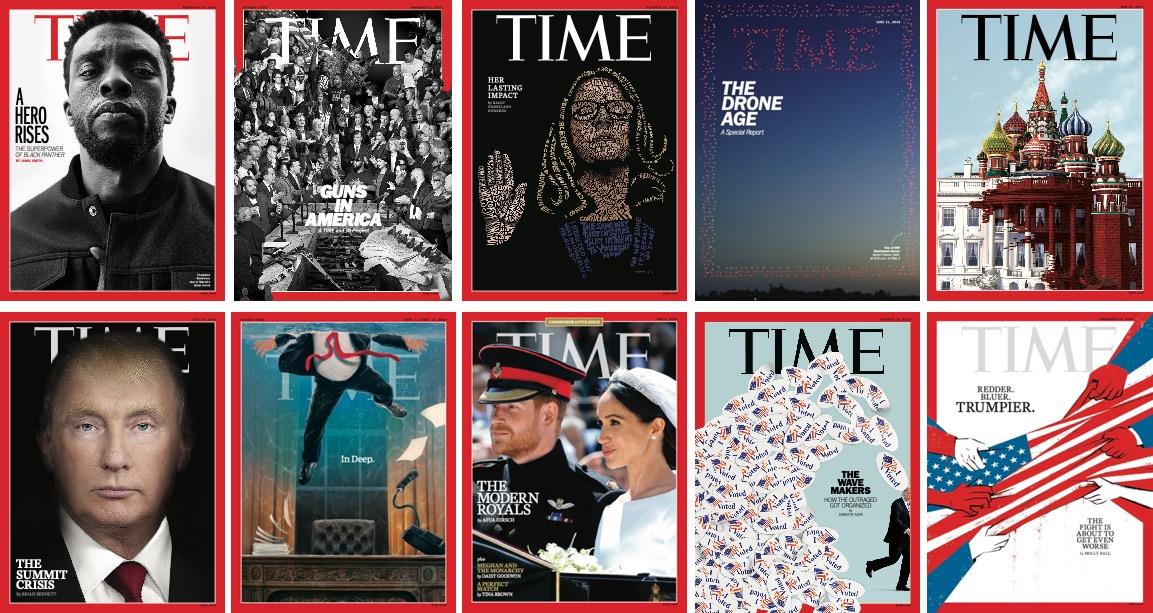This image is a collage of 10 distinct Time Magazine covers arranged in two rows of five columns. The top row features the following covers from left to right: Chadwick Boseman, "Guns in America" with a black and white image of people, an illustrated cover depicting Ketanji Brown Jackson being sworn in as a Supreme Court Justice titled "The Lasting Impact," "The Drone Age" showcasing multiple drones in the sky, and a composite illustration blending the White House with a foreign building, possibly an Indian or Saudi Arabian temple. The bottom row begins with a cover photo of Donald Trump, followed by an illustration titled "In Deep" showing a figure in a suit submerged in water with a desk below him. Next is "The Modern Royals" featuring Meghan Markle and Prince Harry, and an image composed of "I Voted" stickers forming wave patterns labeled "The Movemakers." The final cover in the bottom row displays a tug-of-war scene with multiple hands pulling at an American flag under the title "Redder, Bluer, Trumpier."